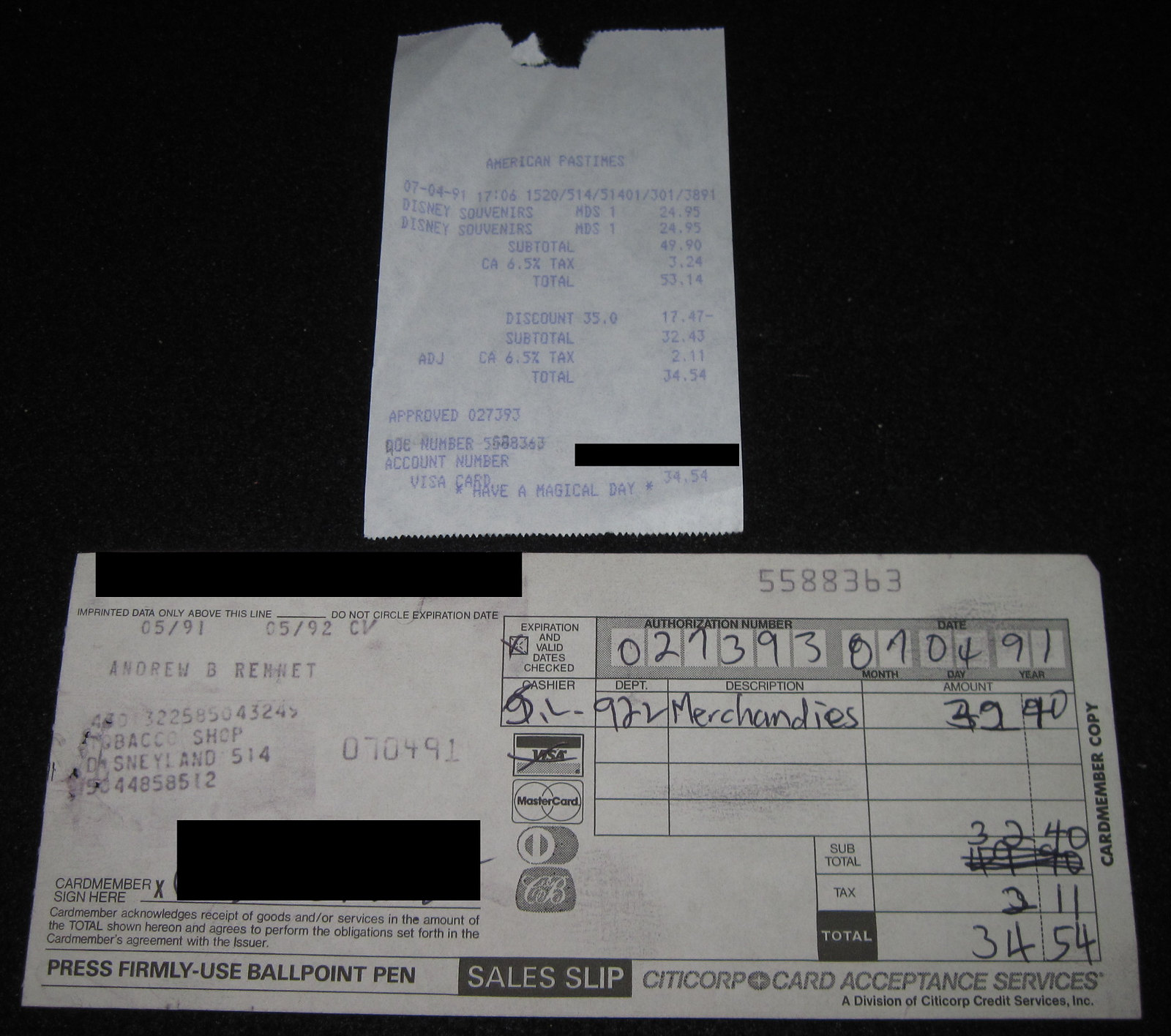In a photograph taken indoors under dim lighting against a black surface, two different sales receipts are displayed. The top receipt, centered in the image, is from American Pastimes and features blue digital printing on white paper. This regular till slip details the purchase of Disney souvenirs priced at $24.95 each, totaling $53.14. It ends with the cheerful message, "Have a magical day." Below it runs an old-school, white credit card receipt, sprawling horizontally across the bottom of the picture. This carbon copy, imprinted with card details from a manual swipe, names the customer as Andrew R. Rennett. Issued from the tobacco shop at Disneyland, it shows a total of $34.54, noted by Citicorp Card Acceptance Services. The entire scene is rendered in shades of black, white, and gray.